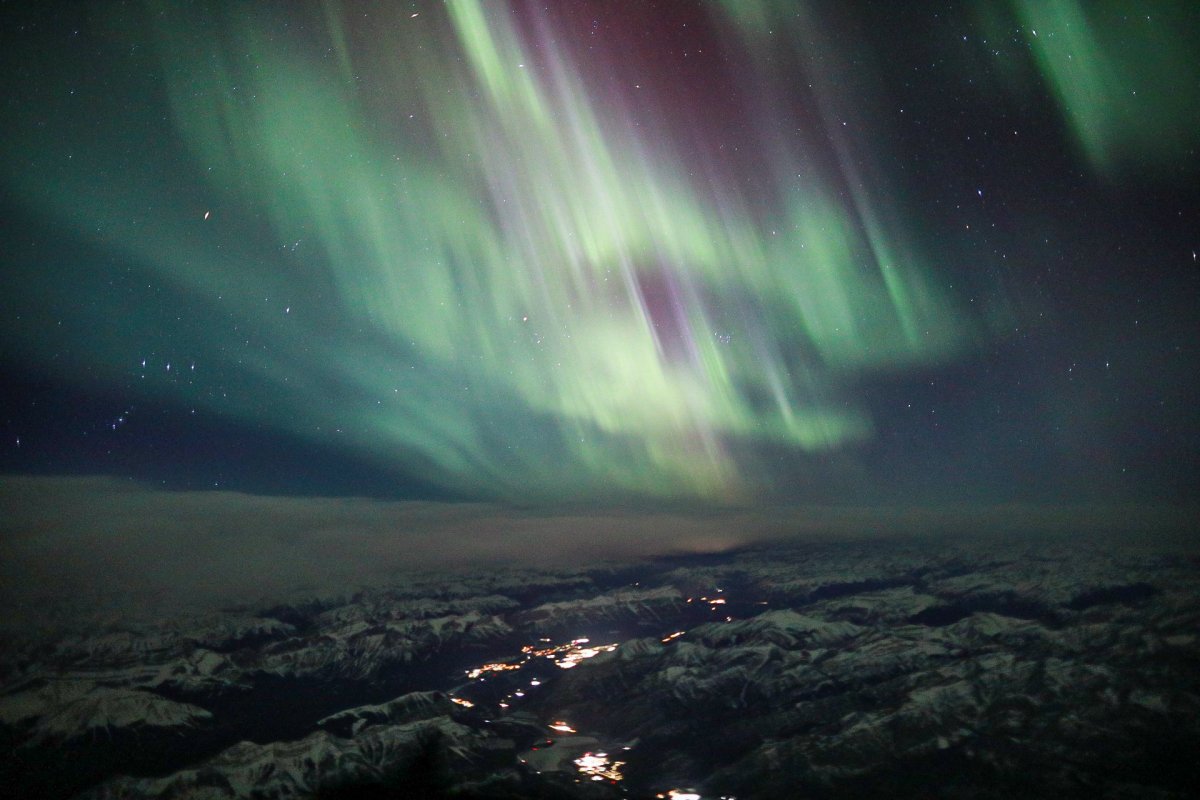In this mesmerizing, night-time photograph, the scene unfolds with the aurora borealis painting the sky in ethereal shades of violet, green, and yellow, forming parallel walls of light. The vibrant purple dominates the middle top, while green hues spread across the middle to the left, with a bit of green shine gracing the upper right. The night sky is dotted with countless stars, their white specks glittering amid the auroras.

Below this celestial dance, the ground extends across roughly a third of the image, showcasing a stark, mystique landscape. The terrain appears gray, black, and bluish, with a volcanic aura. In the middle towards the bottom, a shiny stream weaves through crevices and cracks, suggesting bubbling lava beneath. Further down, a brownish smog or fog-like formation adds to the mysterious ambiance, contrasting the luminous sky above.